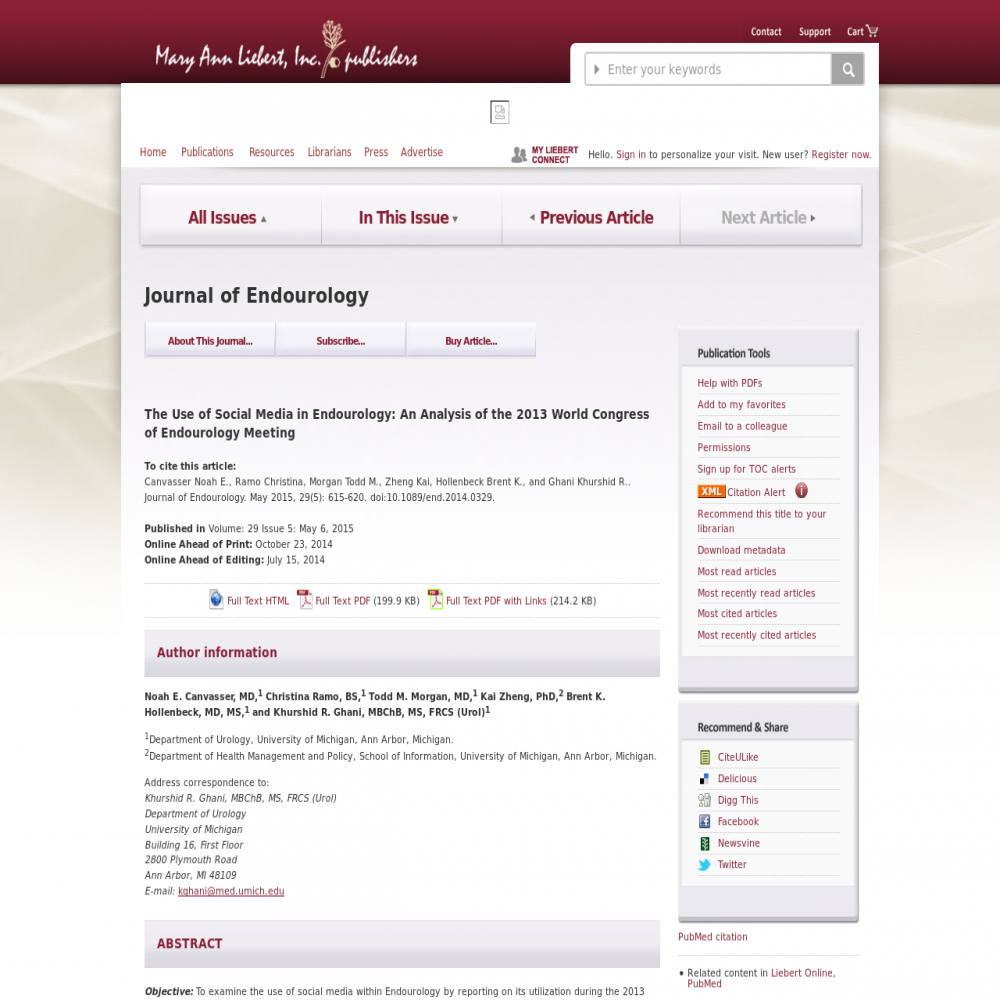This screenshot captures a well-organized and professional-looking website for Marion I. Leibert Inc. Publishers. The webpage features a prominent horizontal rectangle across the top, rendered in a purplish-maroon color, with the publisher's name elegantly displayed in white font. In the right corner of this banner, options for 'contact support' and a shopping cart icon are also in white font. Adjacent to this is a search bar labeled 'Enter your keywords' in gray, equipped with a white magnifying glass icon within a gray square.

The background of the site is primarily white, offering a clean canvas for the black font used for the main content. The navigation tabs, which are a dark maroon color, add a cohesive element to the site's color palette. On the right side of the page, there are publication tools and help links organized into two vertical sections; the first a taller rectangle and the second a more square-shaped one directly beneath it.

Central to the webpage is the 'Journal of Enderology' header in black font, under which three tabs in maroon font offer quick links to 'About this Journal,' 'Subscribe,' and 'Buy Article.' Additional download links also appear in maroon within this section. The layout of the page is balanced and easy to navigate, with the highlighted tab 'Next Article' clearly marked in gray. To the left, more maroon links direct readers to 'Previous Article,' 'In This Issue,' and 'All Issues.' Overall, the website exudes professionalism and readability, ensuring a seamless user experience.